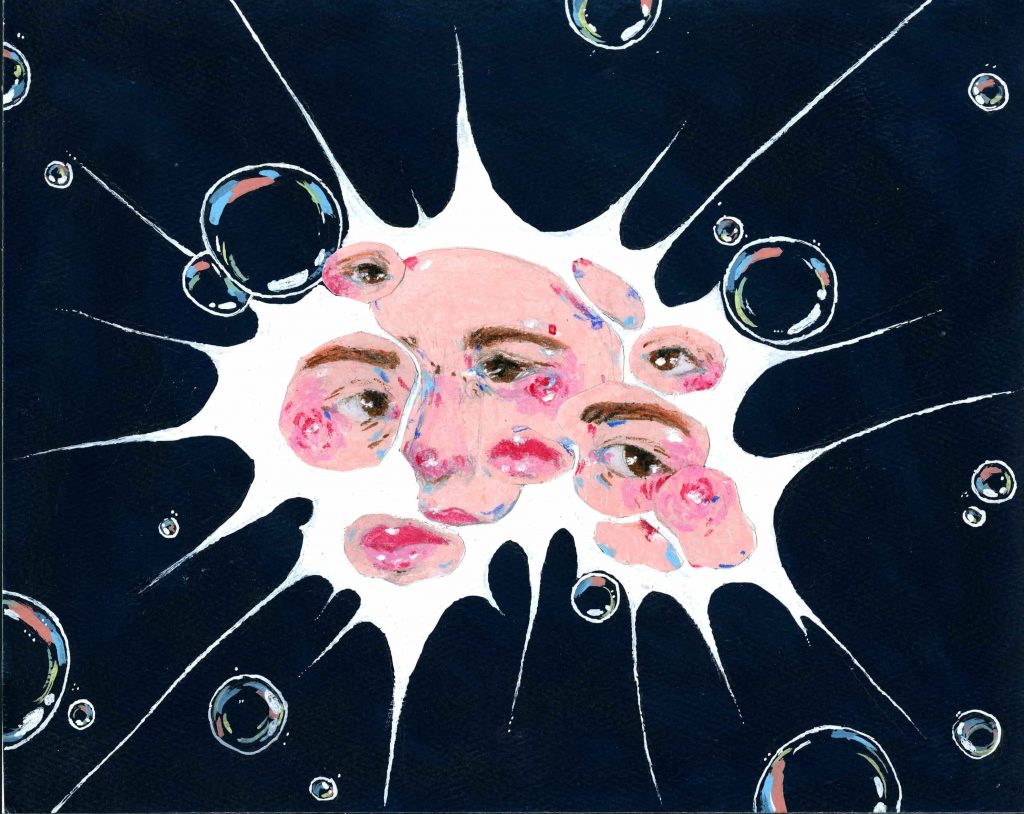The image depicts a surreal and artistic representation created with pencils or a digital medium. The background is a deep, almost black or dark blue color. At the center of the image, there is a striking white splash that looks like splattered paint. This splash is the central focus and extends outward with streaks in all directions. Embedded within this white splash are fragmented parts of a human face. The segments include multiple eyes, lips, and portions of the face, each appearing in various places throughout the splash. The facial features are rendered with natural tones—pink skin, brown eyebrows, and red lips. Surrounding the splash, the dark background is dotted with bubbles, which contain hints of blue, pink, and white hues, adding to the dreamy, collage-like effect of the artwork.